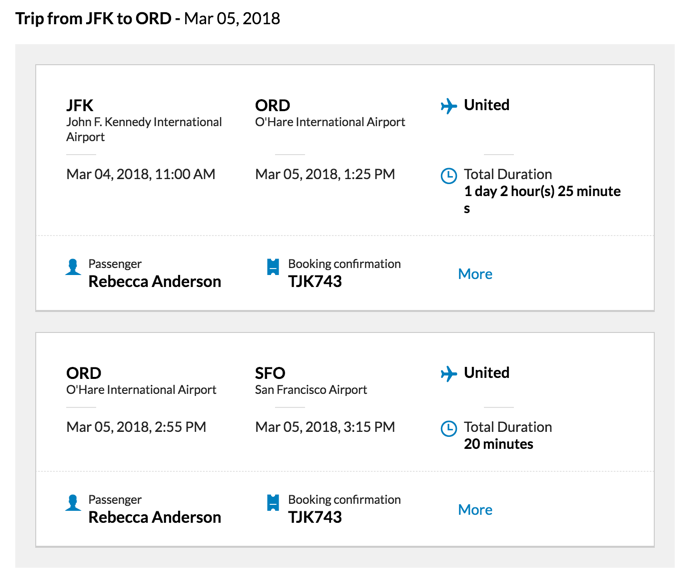**Detailed Itinerary for Rebecca Anderson's Trip:**

**Header:**
- **Trip from JFK to ORD - MAR 05, 2018**

**First Section:**

1. **Departure Information:**
   - **Airport:** JFK (John F. Kennedy International Airport)
   - **Date:** March 4, 2018
   - **Time:** 11:00 a.m.
   - **Passenger:** Rebecca Anderson

2. **Arrival Information:**
   - **Airport:** O'Hare International Airport (ORD)
   - **Date:** March 5, 2018
   - **Time:** 1:25 p.m.
   - **Booking Confirmation:** TJK743

3. **Flight Details:**
   - **Airline:** United Airlines
   - **Image:** Airplane icon
   - **Total Duration:** 1 day, 2 hours, 25 minutes

**Second Section:**

1. **Departure Information:**
   - **Airport:** O'Hare International Airport (ORD)
   - **Date:** March 5, 2018
   - **Time:** 2:55 p.m.

2. **Arrival Information:**
   - **Airport:** San Francisco Airport (SFO)
   - **Date:** March 5, 2018
   - **Time:** 3:15 p.m.

3. **Flight Details:**
   - **Airline:** United Airlines
   - **Image:** Blue airplane icon
   - **Total Duration:** 20 minutes

**Passenger and Booking:**
- **Passenger:** Rebecca Anderson
- **Booking Confirmation:** TJK743

This structured itinerary consolidates Rebecca Anderson's travel details, offering clarity on departure and arrival times, airports, and flight durations.